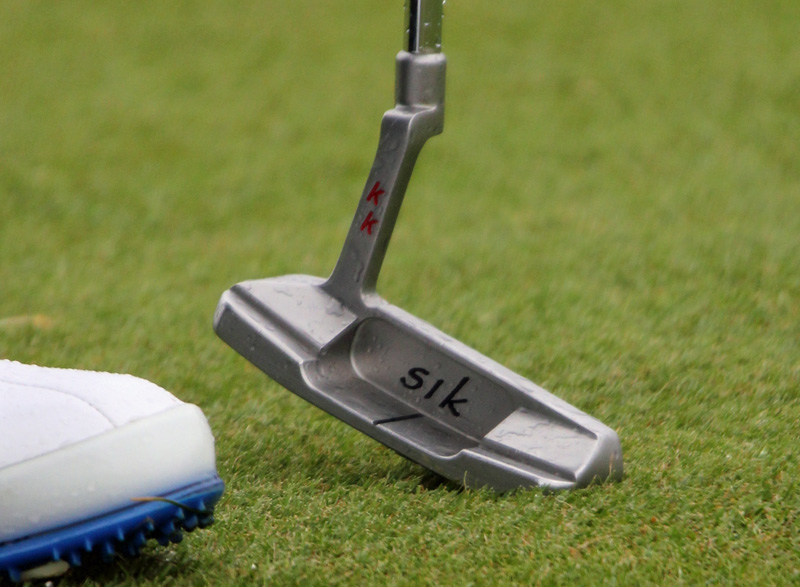The image is a close-up shot of a silver golf putter head resting on very short, green grass, likely on a golf course. The putter head is rectangular with a recessed center that displays black letters spelling "S-I-K". At the junction where the head meets the handle, the letters "K-K" in red are visible. The putter handle is pointing straight upwards. In the bottom left corner of the shot, the toe section of a golfer's shoe is partially visible. The shoe is predominantly white with a white band near the bottom, while the sole is blue with multiple small blue spikes. The scene appears to be taken outdoors, possibly during the day.